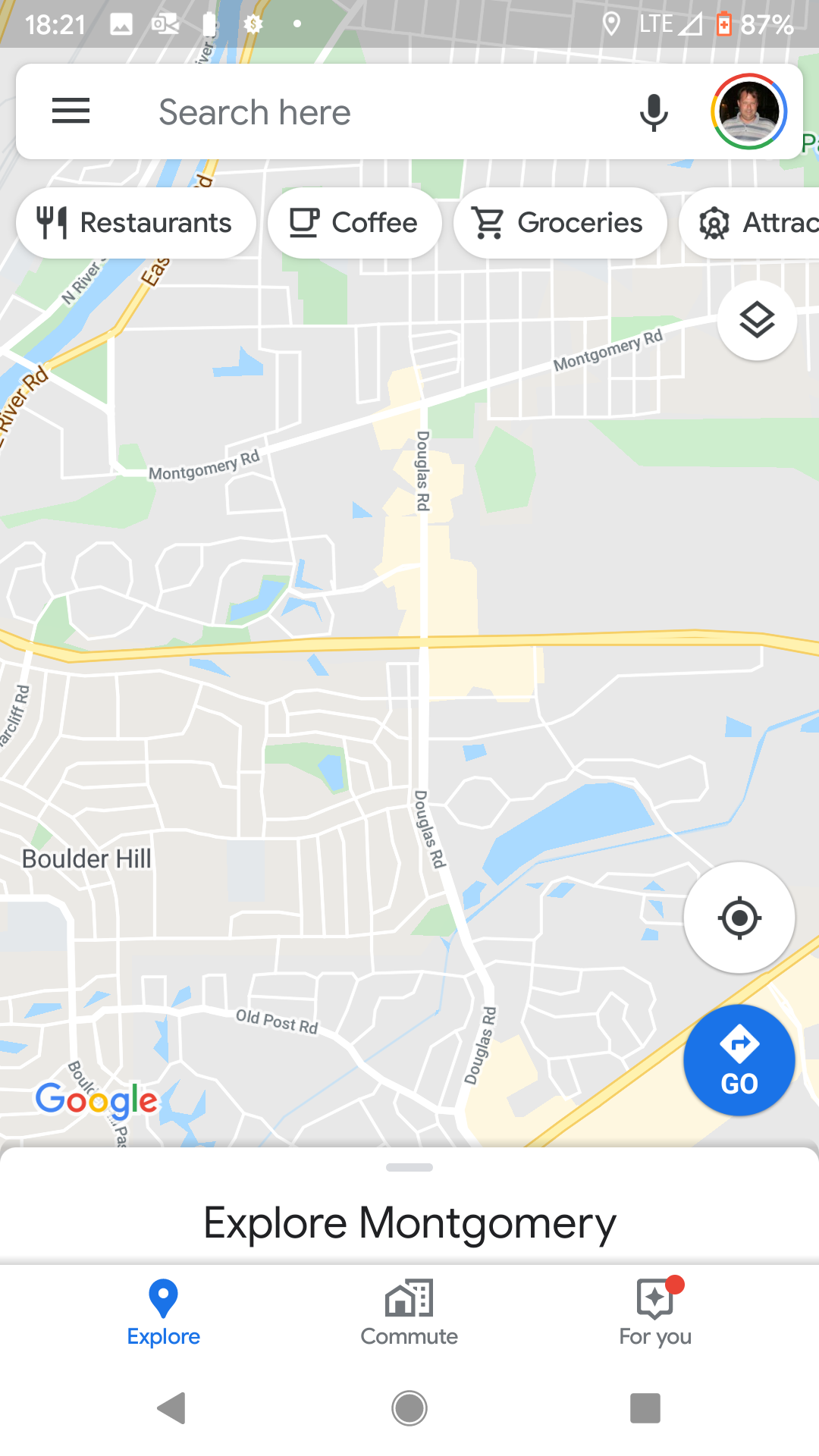This is a detailed screenshot from a Google Maps app on a mobile device. At the very top of the screen, there is a slightly opaque greyed-out bar displaying the mobile phone status information. Notably, the time reads 18:21, and there are four various system icons, one of which indicates a low battery level. Below this bar, there is a search field labeled "Search here" equipped with a microphone icon to its right, and further to the right, the user's profile icon. Beneath this, there are pill-shaped category icons for quick searches, including options like "Restaurants," "Coffee," "Groceries," and "Attractions."

Displayed prominently in the middle section of the screen is the map view of an area named Boulder Hill. The map style appears cartographic, distinguishing it from a terrain or satellite view. Key roads such as Montgomery Road, Douglas Road, Old Post Road, and Boulder Hill are visible. The area also features a small pond or lake, several additional minor bodies of water, and a river situated towards the top left-hand corner of the screen. 

At the bottom of the map, there is a section labeled "Explore Montgomery" with three icons for different functionalities: exploring the area, managing commutes, and additional clickable options.